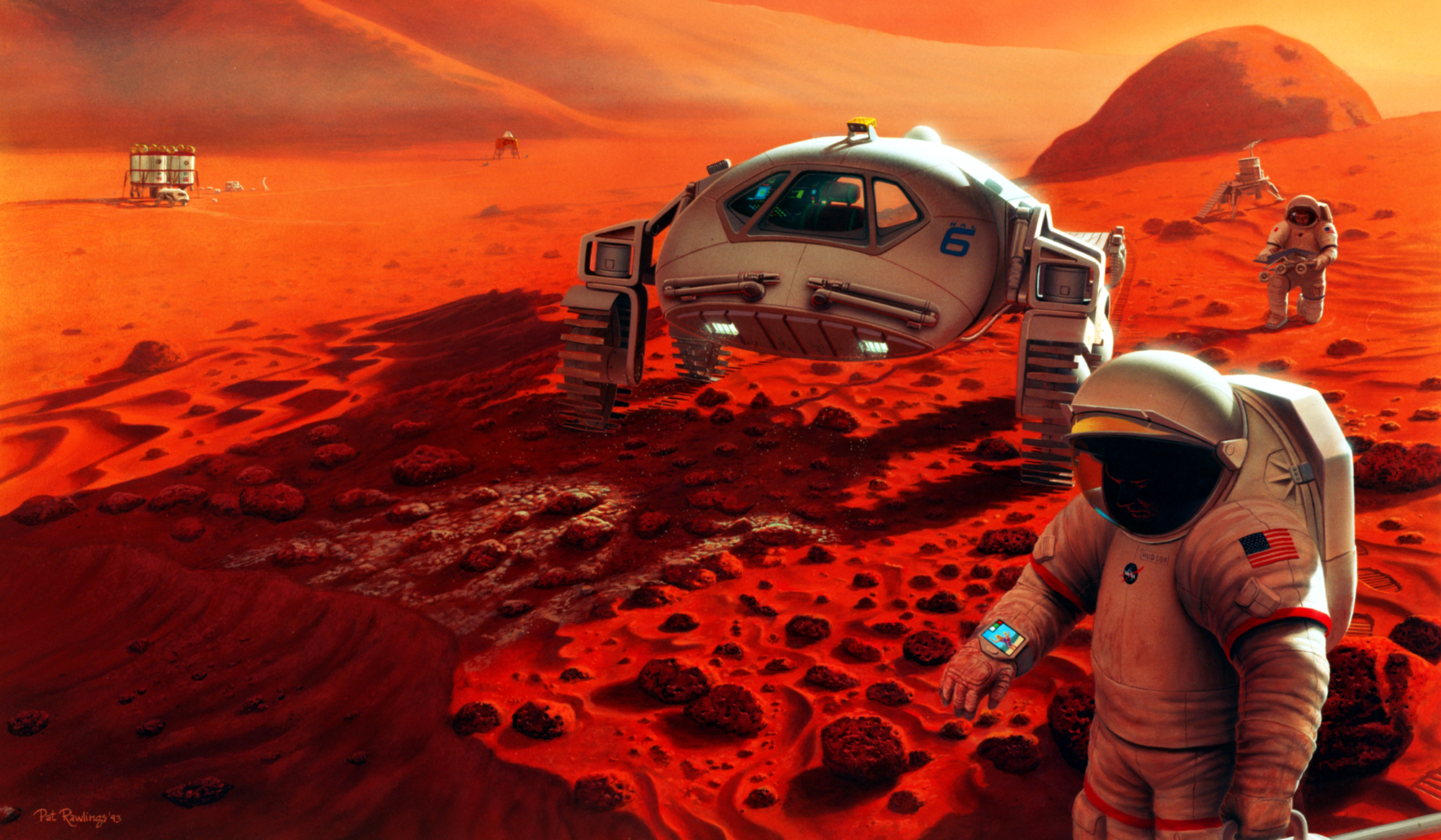This is a detailed color sketch by Pat Rawlings from 1993, depicting life on Mars. The image features two astronauts in U.S. NASA space suits on the rocky red surface of the planet, identifiable by its red rocks, hills, and mountains. The astronaut in the foreground is standing and looking at a communication device on his wrist, with the American flag and NASA symbol visible on his suit. Behind him, another astronaut is kneeling, possibly taking surface samples. Central to the scene is a modern, high-riding space rover with large windows and track-like wheels, designed to navigate the challenging Martian terrain. In the background, there is another large robotic machine labeled "number six," which appears to be part of their exploratory equipment. Additionally, a small space station is visible in the left background, hinting at the human presence and activity on the Red Planet.